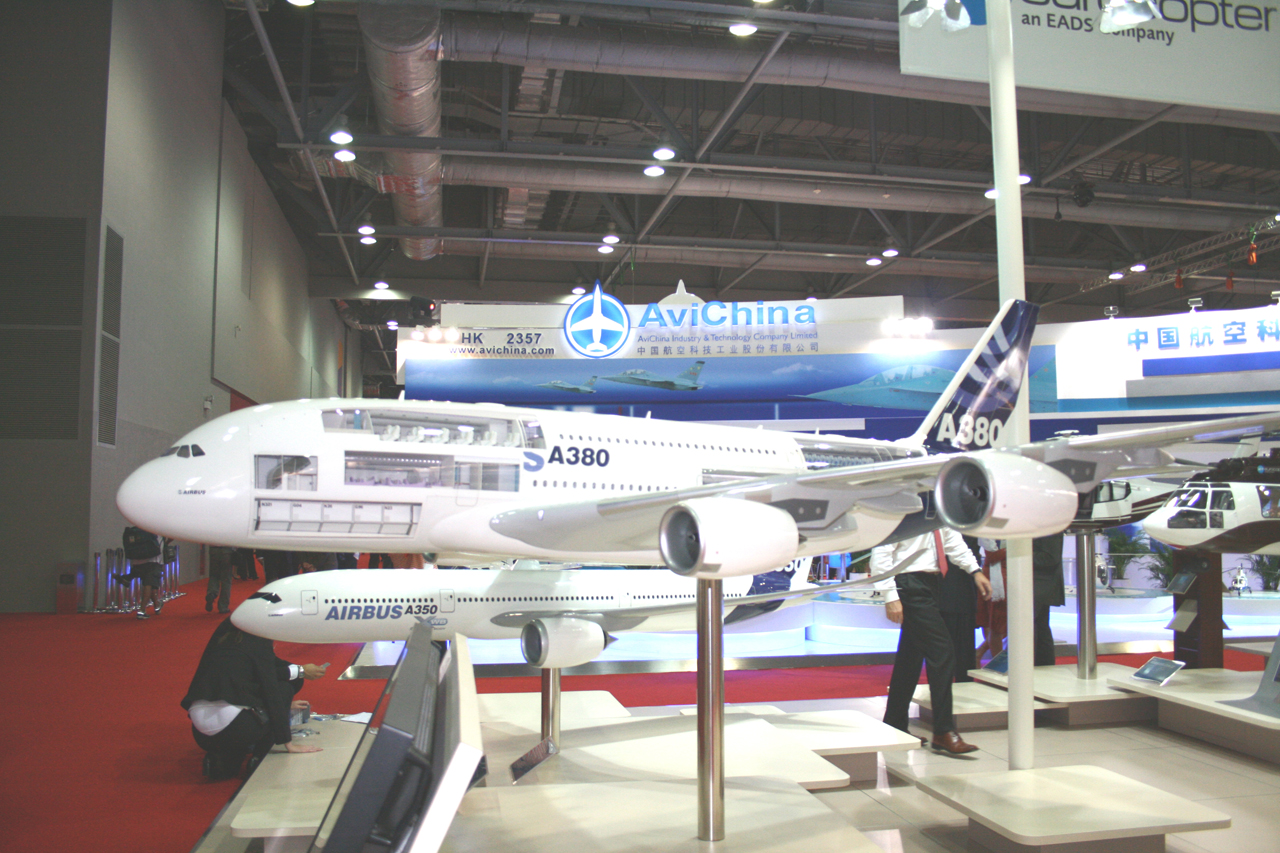The image depicts a detailed exhibition display of two model airplanes at an aerospace museum or convention, prominently marked "AviChina." The setting is an indoor space with visible pipes and lights overhead, and the area is carpeted in red. The largest model airplane in the foreground is identified as an A-380, featuring a distinctive double-decker design with two rows of seating and marked with "SA308." This model has sections exposed through glass panels, showcasing the internal compartments like the passenger area and luggage compartments. Behind it is a smaller Airbus A-350 model, also white with navy and light blue lettering. The scene includes two individuals: one crouching near the Airbus A-350, wearing a black suit, white shirt, and black trousers, and another whose bottom half is visible, dressed in a white shirt with a red tie, black trousers, and brown shoes. The overall ambiance suggests a professional and formal atmosphere, with business professionals present at the exhibit.